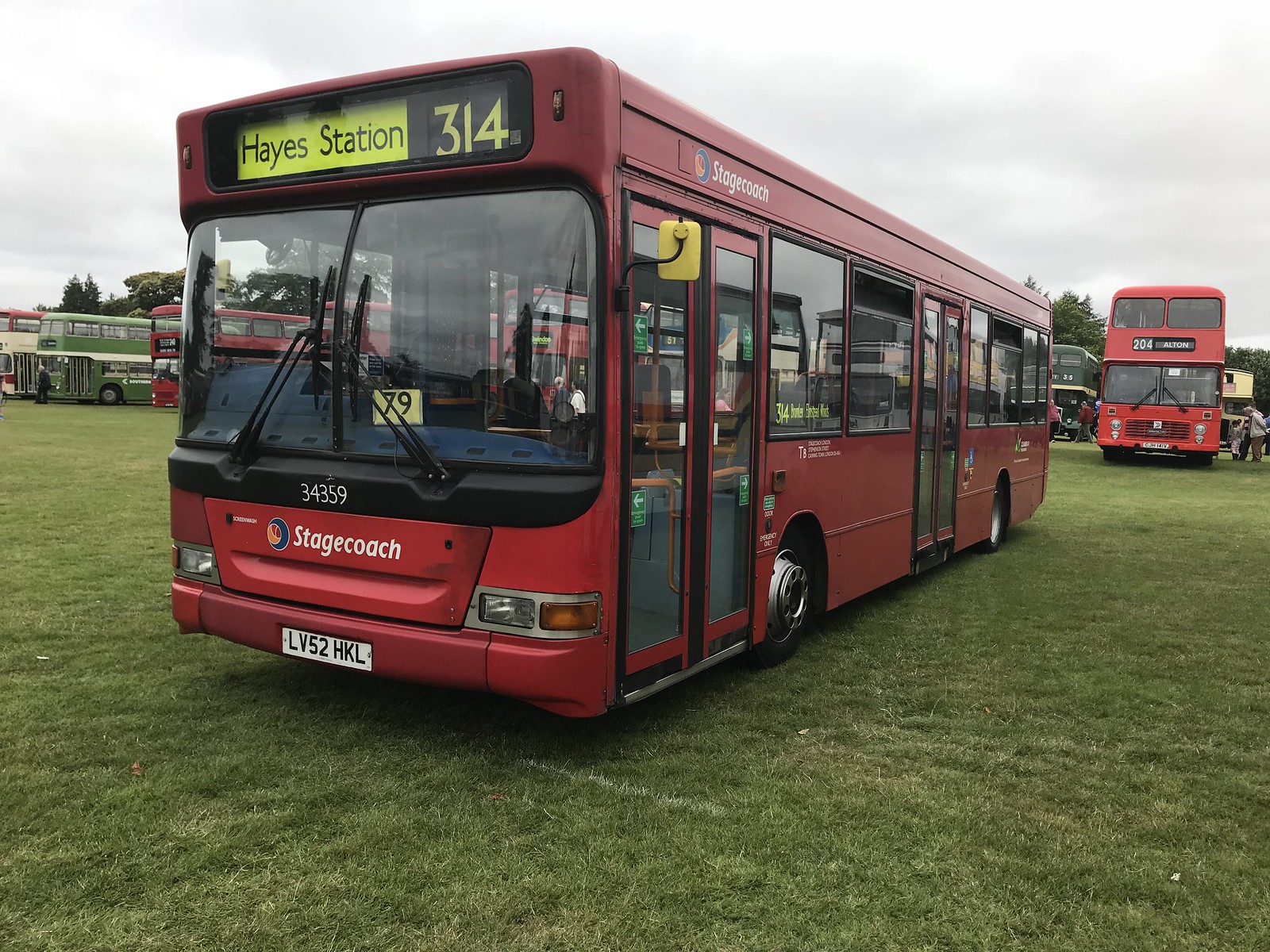The image captures a striking red bus prominently parked on a vibrant green lawn, set against a backdrop of various other buses in different colors and styles, including yellow, green, and iconic double-decker models. This modern red bus, taking center stage in the photograph, is labeled with "Hayes Station 314" in bold, neon-like text on its front display. Below this sign, the logo of its operating company, "Stagecoach," is clearly visible. The bus is equipped with two accordion doors on its right side and expansive windows along its length, providing a sleek, contemporary appearance. The bus features a white license plate reading "LV52 HKL," flanked by clear headlights with adjacent orange blinker lights. Yellow driver's side mirrors can be seen reflecting the surroundings. The other buses in the scene appear to be part of a display or exhibition, all empty inside with their interiors visible through the large windows, underscoring the show-like atmosphere as people meander around, observing the vintage and modern vehicles on display.